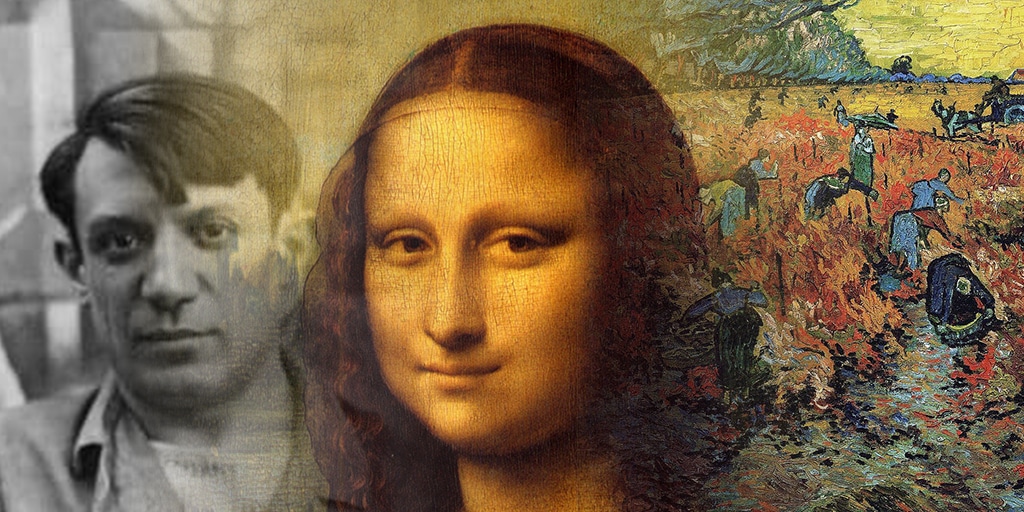The image is a seamless rectangular triptych merging three distinct pieces into a cohesive flow. On the left is a black and white photograph of a Caucasian man in his 30s, seemingly taken in the 1940s or 50s, dressed in working attire. This transitions smoothly into the iconic Mona Lisa at the center, portrayed in her classic, unaltered form. The right side features a vibrant, pastoral scene reminiscent of Van Gogh’s style, depicting people working in a field, possibly harvesting wheat, with a man visible on a wagon. The entire composition is unified with hues of pink, blue, purple, and gray, blending these diverse images into a harmonious array without any harsh separations or borders.